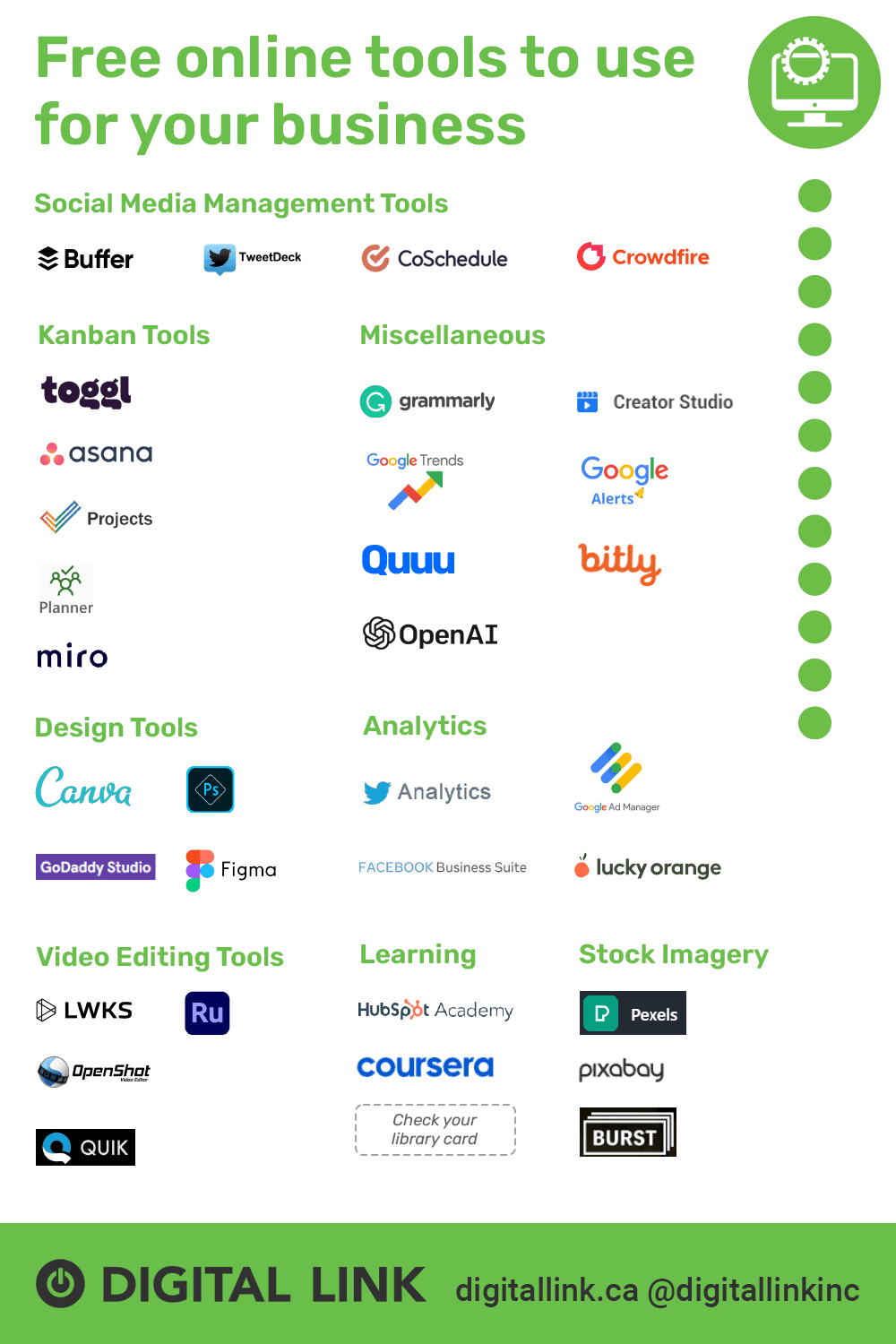This digital advertisement is a clean and informative poster designed to provide business owners with a curated list of free online tools. Set against a crisp white background, the poster's primary color scheme features varying shades of green. 

At the bottom of the advertisement, a green band runs horizontally across the width, adorned with black text that reads "Digital Link." Situated in the bottom-left corner, the logo includes the phrase "Digital Link," accompanied by a power button icon, adding a modern touch. Below the logo, the text "digitallink.ca" and "Digital Link Inc" is displayed.

The header boldly announces, "Free Online Tools to Use for Your Business," effectively capturing attention. Below the header, the poster is divided into several categories that highlight essential tools: Social Media Management Tools, Command Tools, Miscellaneous, Design Tools, Analytics, Video Editing Tools, Learning, and Stock Imagery. 

Each category features logos from various websites and services, making it easy for viewers to identify recommended tools. These logos are organized in a tidy grid layout with distinct rows and columns, ensuring a visually appealing and straightforward presentation.

An infographic element complements the theme, featuring a computer screen with a gear enclosed in a green circle, symbolizing digital efficiency and innovation. Additionally, there's a subtle dotted line pattern running vertically underneath this iconography, adding a touch of sophistication to the overall minimalist design.